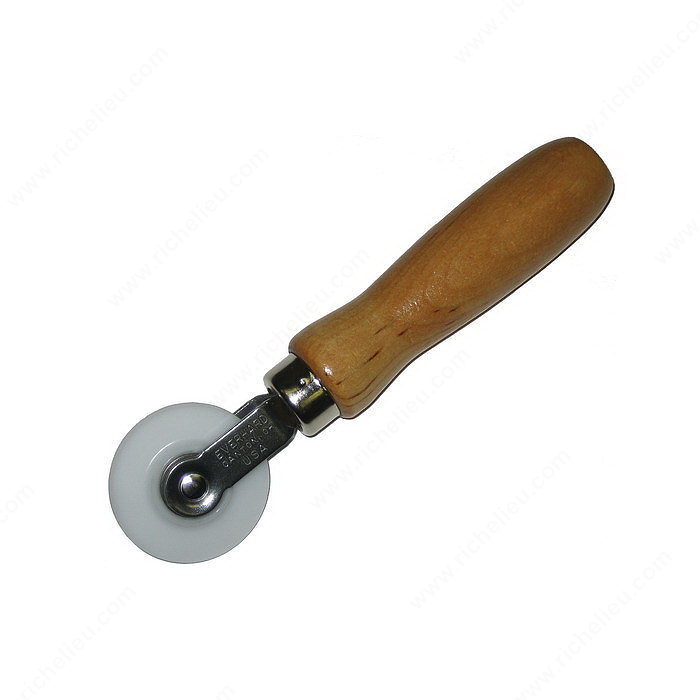This image features a handheld device with a wooden handle and a wheel at one end, resembling a caster. The handle is made of orangish-brown wood with visible grain, reflecting light in places. Attached to this handle with a stainless steel nut is a heavy metal piece engraved with "Everhard Canton Ohio USA". This metal section extends into two forks that hold a white, round wheel, likely made of plastic or glass, giving it the appearance of a roller or dolly part. The entire device is displayed against a plain white background, with the wheel pointing downwards and the handle pointing upwards.